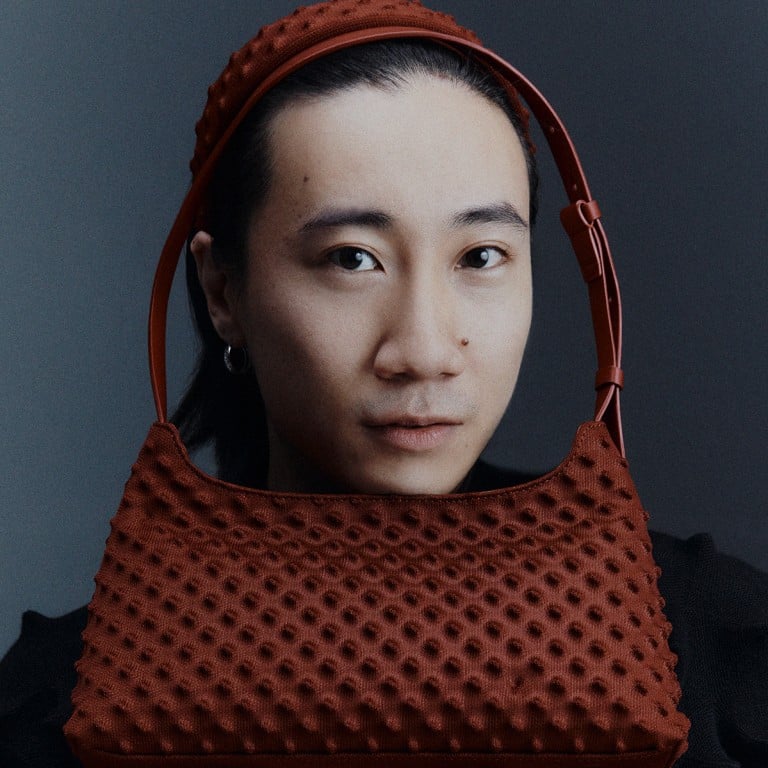In this fashion photograph with a gray background, an androgynous Asian model gazes directly at the camera. The model, with strikingly black hair pulled into a ponytail, bushy black eyebrows, and black eyes, is characterized by a broad nose and a distinctive mole on the left side of their nose. They have pale lips and skin and sport small hoop earrings. Framing their face is a knobby, reddish-brown leather handbag with a smooth, adjustable buckled strap. The handbag, hanging from their forehead with its bottom just beneath their chin, creates a unique visual contour against their features. They are dressed in a black top, which blends seamlessly into the dark, minimalist background, emphasizing the texture and color of the handbag and the serene yet intense expression of the model.